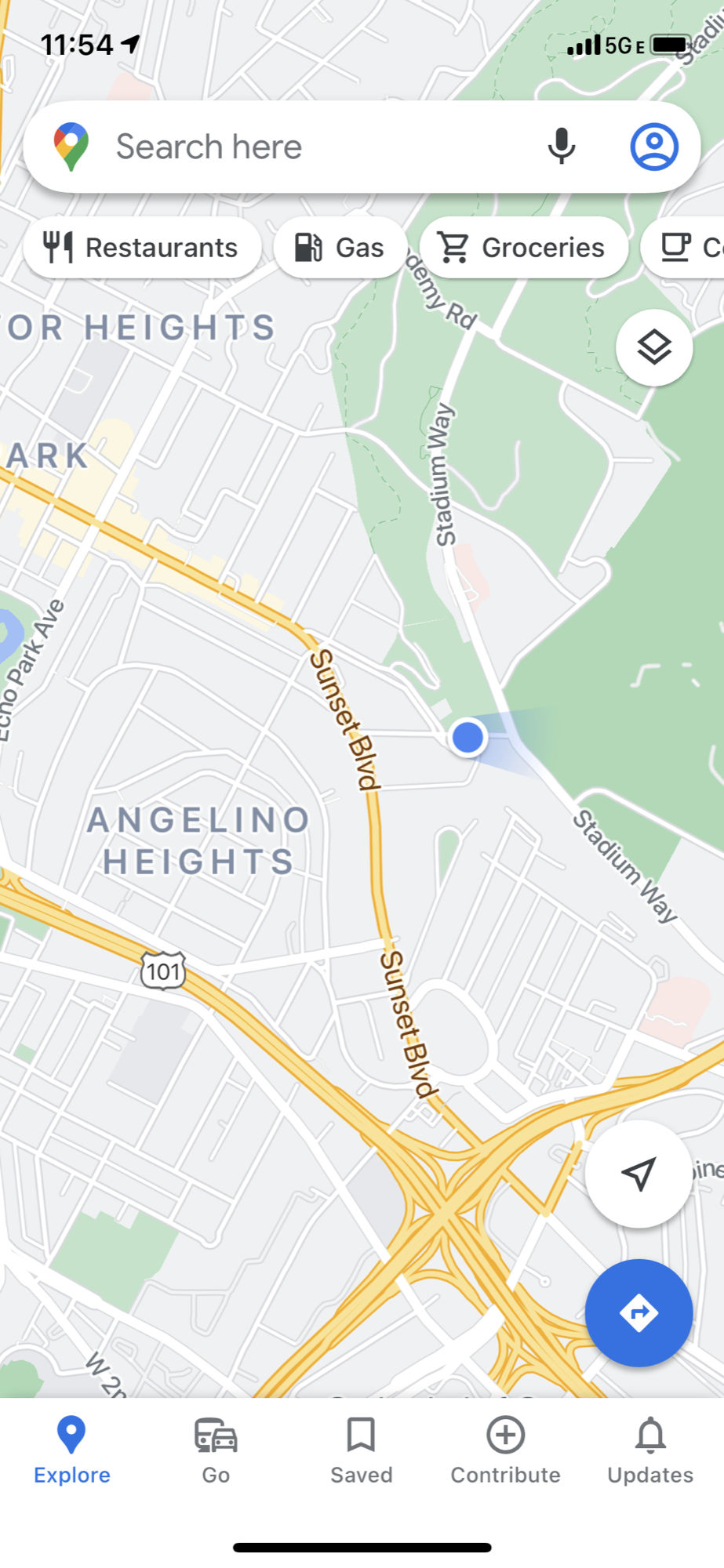Screenshot of a smartphone displaying a detailed map of Los Angeles. At the top of the screen, the time reads 11:54, accompanied by four bars of cellular coverage, indicating a 5G connection, and a full battery icon. Just below, there is a Google search bar with the prompt "Search here," featuring a microphone icon and a user profile icon to the right.

Beneath the search bar are quick access icons for various categories: "Restaurants" marked by a fork and knife icon, "Gas" represented by a gas pump icon, "Groceries" symbolized by a shopping cart icon, and "Coffee" indicated by a coffee cup icon.

The map prominently highlights Sunset Boulevard in orange, and notable locations such as Stadium Way, Angeleno Heights, and Echo Park Avenue are visible. In the bottom right corner, there are two icons: a white circle with a black-outlined arrow pointing diagonally up and to the right, and a blue circle with a white diamond shape in the center, featuring a blue arrow pointing to the right.

At the very bottom of the screen, a navigation bar displays options: "Explore," which is currently highlighted, along with "Go," "Saved," "Contribute," and "Updates."